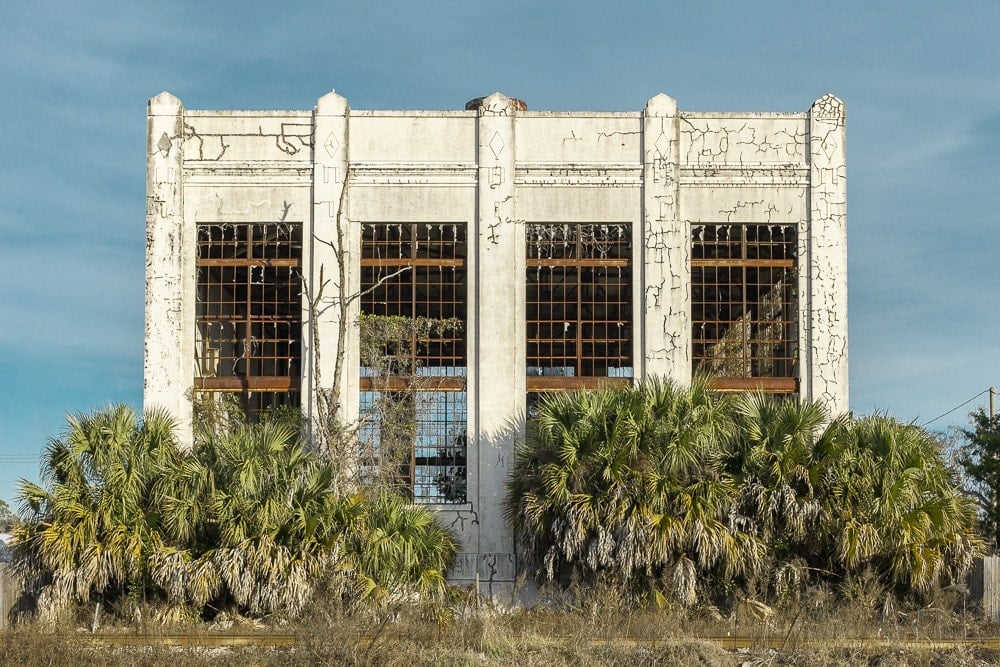The image captures a derelict, old, and abandoned concrete building, possibly located somewhere in Asia, set against a light blue sky with wispy clouds. The exterior white stucco is heavily chipped, cracked, and peeling, revealing years of neglect. Large, overgrown palm bushes flank the building on the left and right, and smaller shrubs with bare, deteriorating bases fill the area in front. The building’s weathered facade features windows now devoid of glass, merely skeletal metal frames rusting away, reminiscent of giant chicken wire. Projections resembling columns separate these window spaces. Through the missing windows, you can see the interior's dark, empty expanse. A telephone pole with intersecting lines can be seen at the bottom right corner, enhancing the scene's sense of desolation.